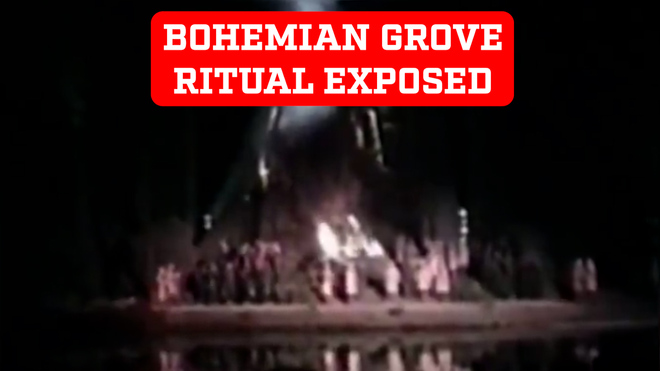The image appears to be a still shot or title card from a YouTube video or television show, featuring the words "Bohemian Grove Ritual Exposed" prominently displayed in large white capital letters on a bright red background at the top and centered. The rest of the image is grainy, overexposed, and primarily black, making it difficult to discern specific details. It depicts a blurry group of humanoid figures, some in light-colored and others in dark-colored clothing, standing around a fire near a shoreline, with reflections visible on the water. The scene appears to be taken at night, heightening the mysterious and ominous atmosphere, possibly intended to evoke curiosity or concern about the purported Bohemian Grove ritual.